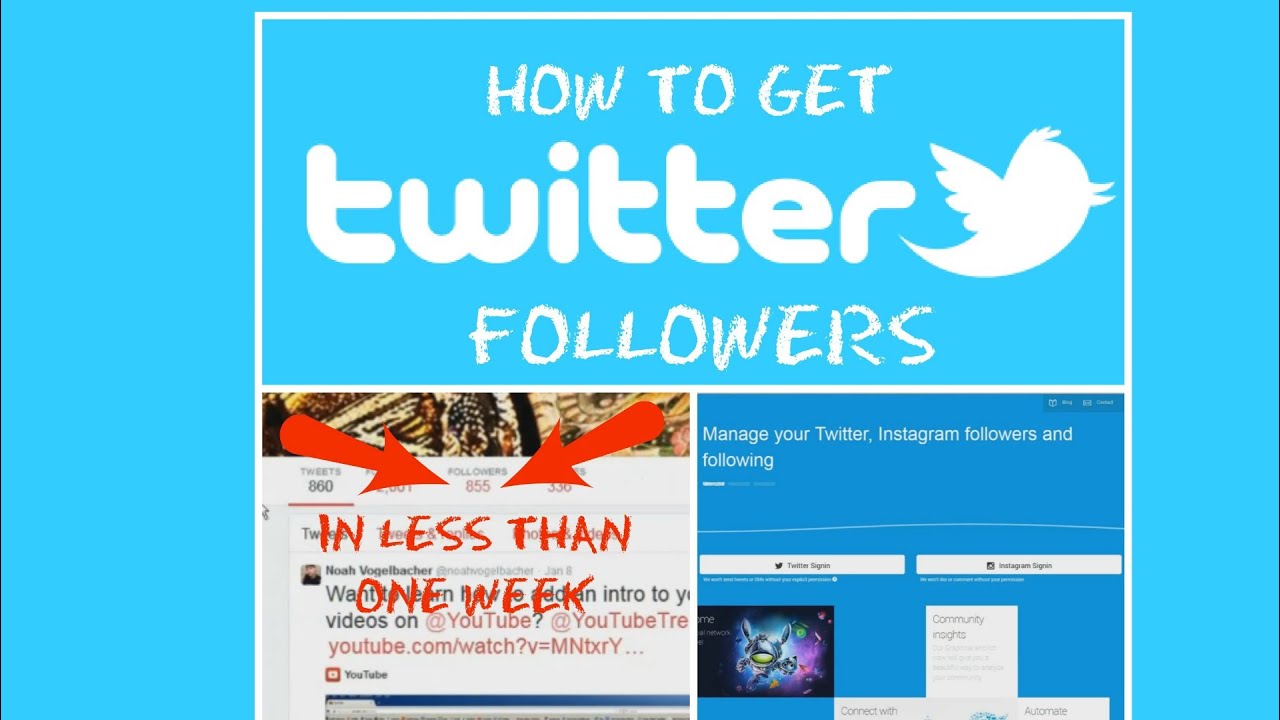This is a detailed and cleaned-up caption for the described image:

---

The screenshot features a promotional webpage focused on e-digital marketing. The main headline, prominently displayed in large letters alongside the Twitter logo, reads: "How to Get Twitter Followers in Less Than One Week." Below this main headline, a visual element includes two red arrows pointing towards a follower count of "855," emphasizing rapid growth. An overlay in a handwritten-style font reinforces the promise: "In less than one week." On the right side of this promotional message, there is a header stating: "Manage Your Twitter and Instagram Followers and Following." The webpage has a light blue background, consistent with Twitter's branding, highlighting the site's specialized marketing services aimed at increasing social media followers efficiently.

---